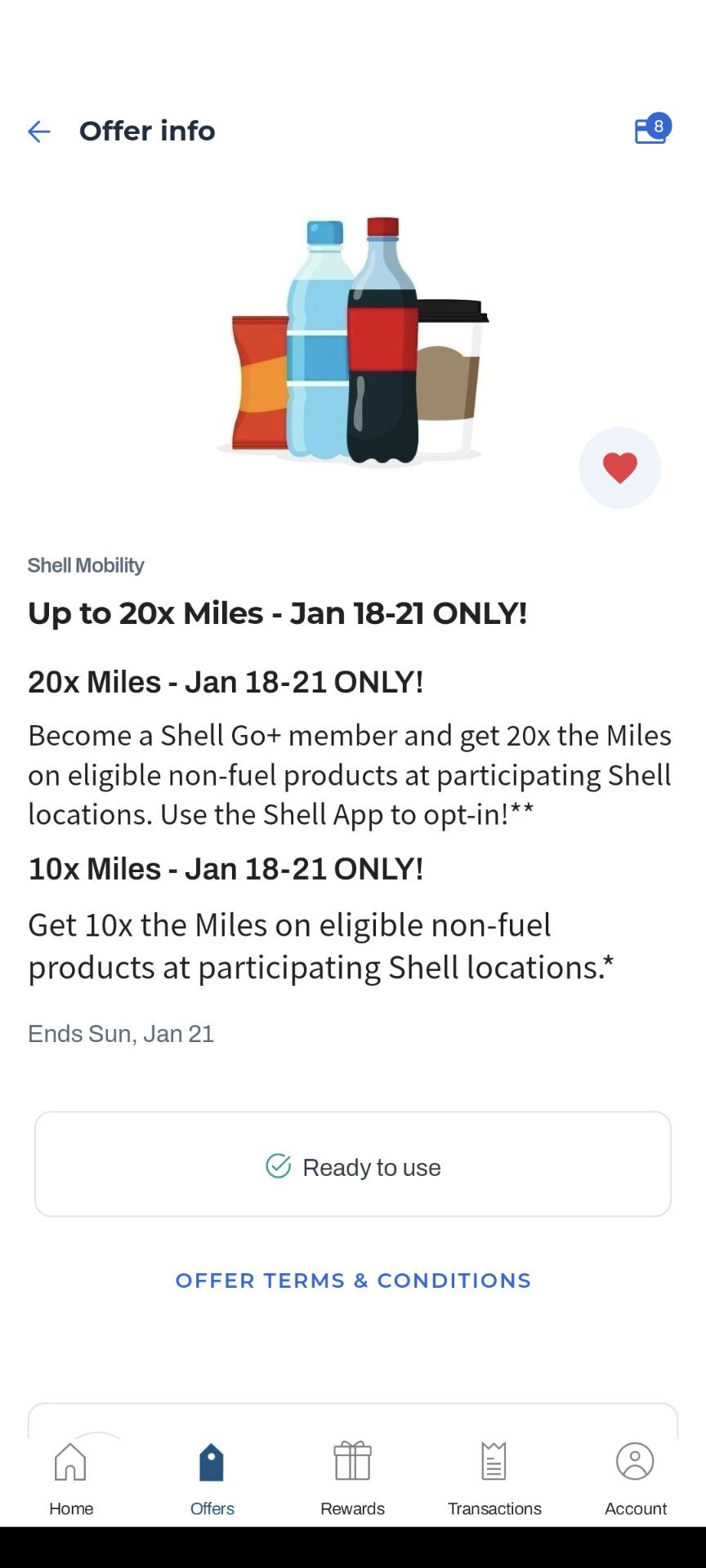The image is a screenshot of an email titled "Offer Info", with a back button highlighted in blue at the top-left corner. On the top-right, there is an icon indicating the user has eight unread emails. The main portion of the email displays several graphic images, including a generic Coca-Cola bottle with a red label and cap, a blue liquid-filled water bottle with a blue and white label and blue cap, a red chip bag with an orange label, and a coffee cup featuring a black lid, white cup, and brown sleeve. Adjacent to these images, a heart-shaped logo accompanies the text: "Shell Mobility - Up to 20X Miles. January 18th through 21st Only". The caption promotes a special offer where Shell Go Plus members can earn 20 times the miles on eligible non-fuel purchases at participating Shell locations. The offer is valid through the specified dates, and members are encouraged to use the Shell app to log in and take advantage of the promotion.